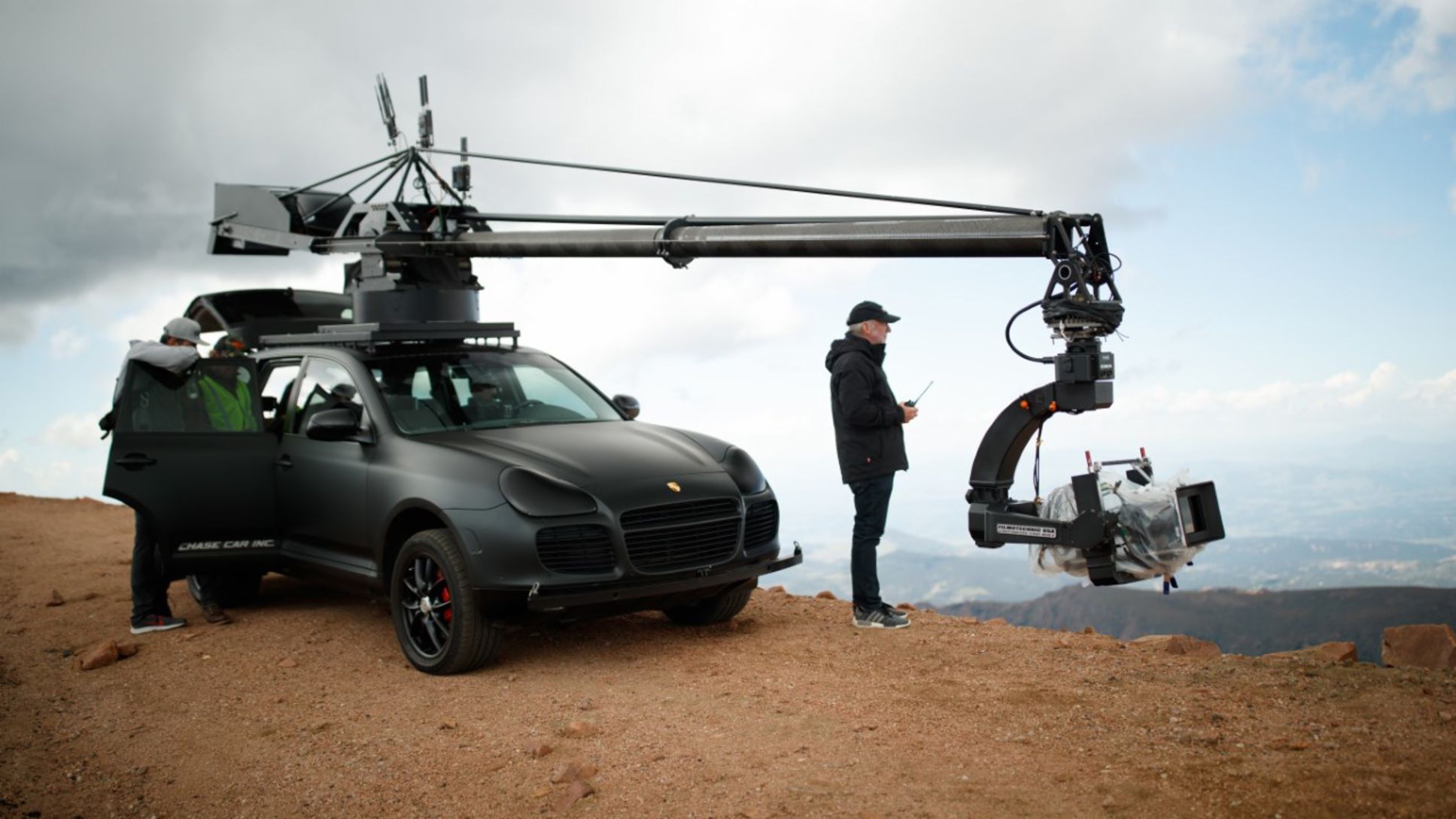The image depicts a dark gray, matte-finish SUV, possibly a Porsche, positioned on the very edge of a high, sandy cliff with a partly cloudy sky above, showing hues of white and light blue. The SUV is equipped with an elaborate camera rig mounted on its roof, which includes a large, flexible boom arm extending out to the front of the vehicle. Attached to the end of this boom is a sizable camera, notable for its big square lens, indicating the setup is likely for movie-making. The scene includes three men: one near the camera, dressed in a jacket and dark-colored cap, possibly holding a remote control or a device with an antenna; and two others by the open rear passenger door, one wearing a light-colored vest and a cap. Within the wheel well of the SUV, through the spokes of the rear tire, something red is visible. The setting is an expansive, almost barren dirt landscape with hints of green, set against a backdrop of distant hills and mountains.